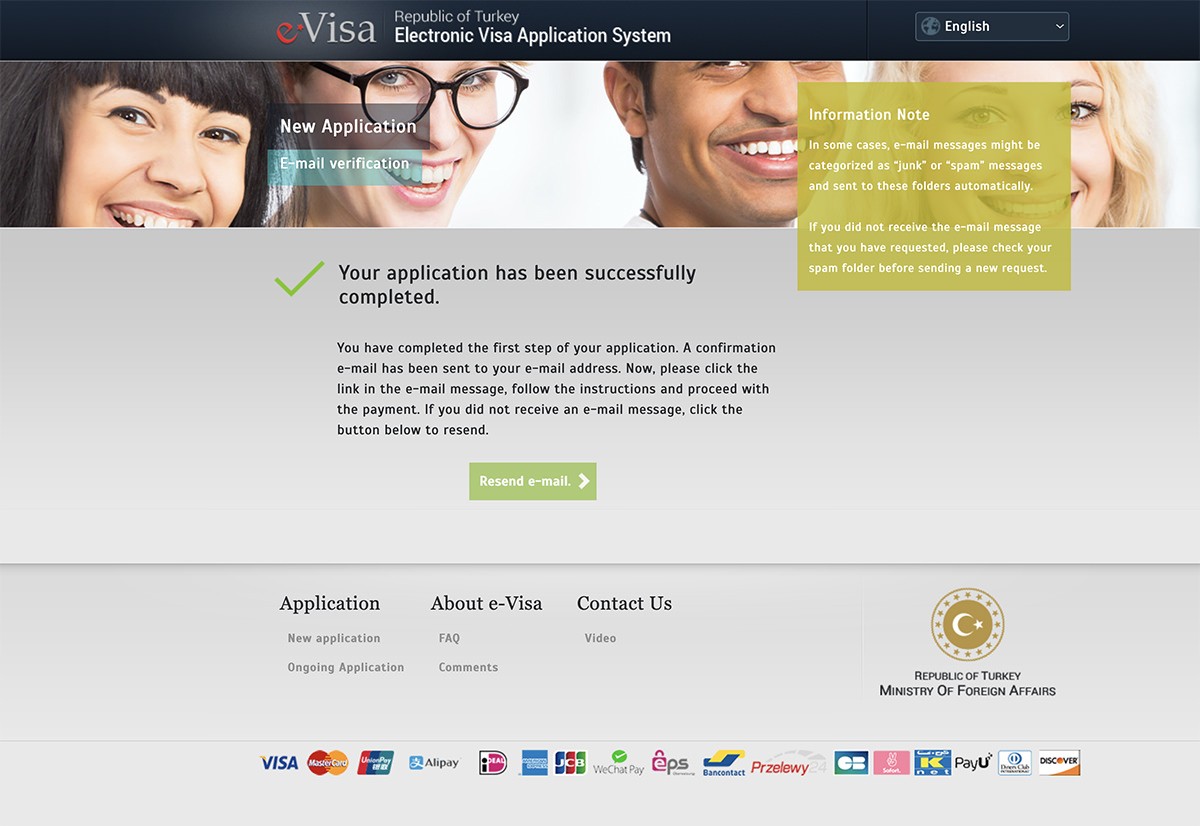This image is a screenshot of a website, slightly wider than it is tall. At the top is a horizontal banner taking up about 5-10% of the image's height. Featured on the left side of the banner is a logo for "eVisa," with the "E" in red, tilted to the left, and "Visa" in gray. Next to the logo, aligned to the right, are the words "Republic of Turkey" in white text, followed by "Electronic Visa Application System." 

On the upper right corner of the banner, there is a dropdown box with a globe icon indicating language options, and it currently displays "English" in white text. Below this banner, occupying approximately 20-25% of the site's height, are images of four individuals representing diverse ethnicities: an Asian person, a Black person, a White man, and a White woman, all smiling. Their faces are partially visible at the top of the screen.

The main content of the website is set against a gray background and is centered within the image. Prominently displayed is a large green check mark, accompanied by black text that reads, "Your application has been successfully completed." This suggests that the webpage serves as a confirmation page for an electronic visa application.